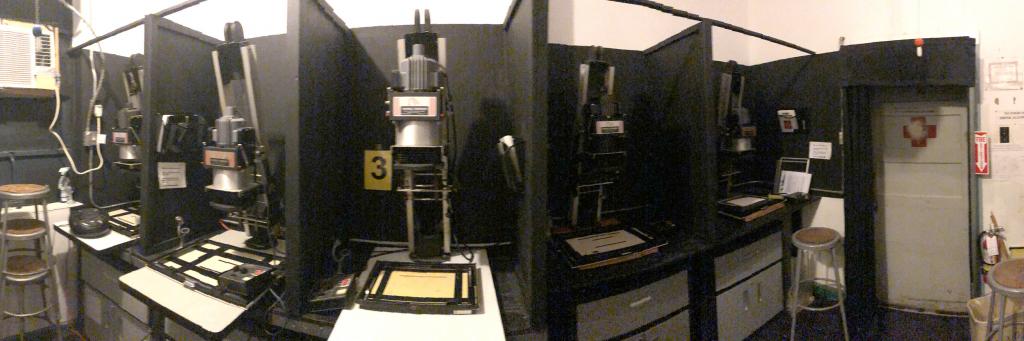The image depicts an indoor work area, resembling an old printing or lithographing factory. It features five identical stations, each equipped with silver and black machines designed to press paper held in a square frame at the bottom. The focal point is Station 3, highlighted with a yellow number. The work area is characterized by its primarily gray and black color scheme, with splashes of red from a health cross on a white door and a red and white fire sign on the right-hand side. The door, centered on a white wall, remains closed. Adjacent to the door, there are cubby holes with black partitions and white drawers beneath each machine. The workspace includes silver barstools with brown tops, positioned on both sides of the room, and a beige garbage can. An air conditioning unit is situated above in the far left corner, where additional stools appear stacked up. A small mail slot is visible on the right, likely used for storing instructions or booklets.